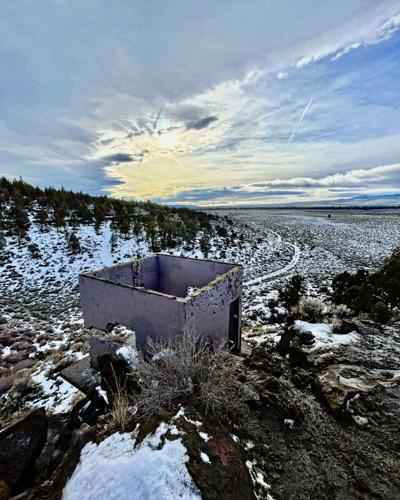The daytime photograph captures a serene, snow-covered landscape adorned with an old, abandoned structure in the middle of nowhere, surrounded by trees and small plants peeking through the melting snow. The focal point of the image is a roofless, gray, concrete building with jagged, broken edges, suggesting it has been worn down by either natural forces or purposeful dismantling. The ground is gently hilly, and in the background, distant mountains rise under a majestic sky painted with wispy clouds blending blues and yellows. The overall scene conveys a sense of desolate beauty and tranquility in a remote, possibly mountainous area.